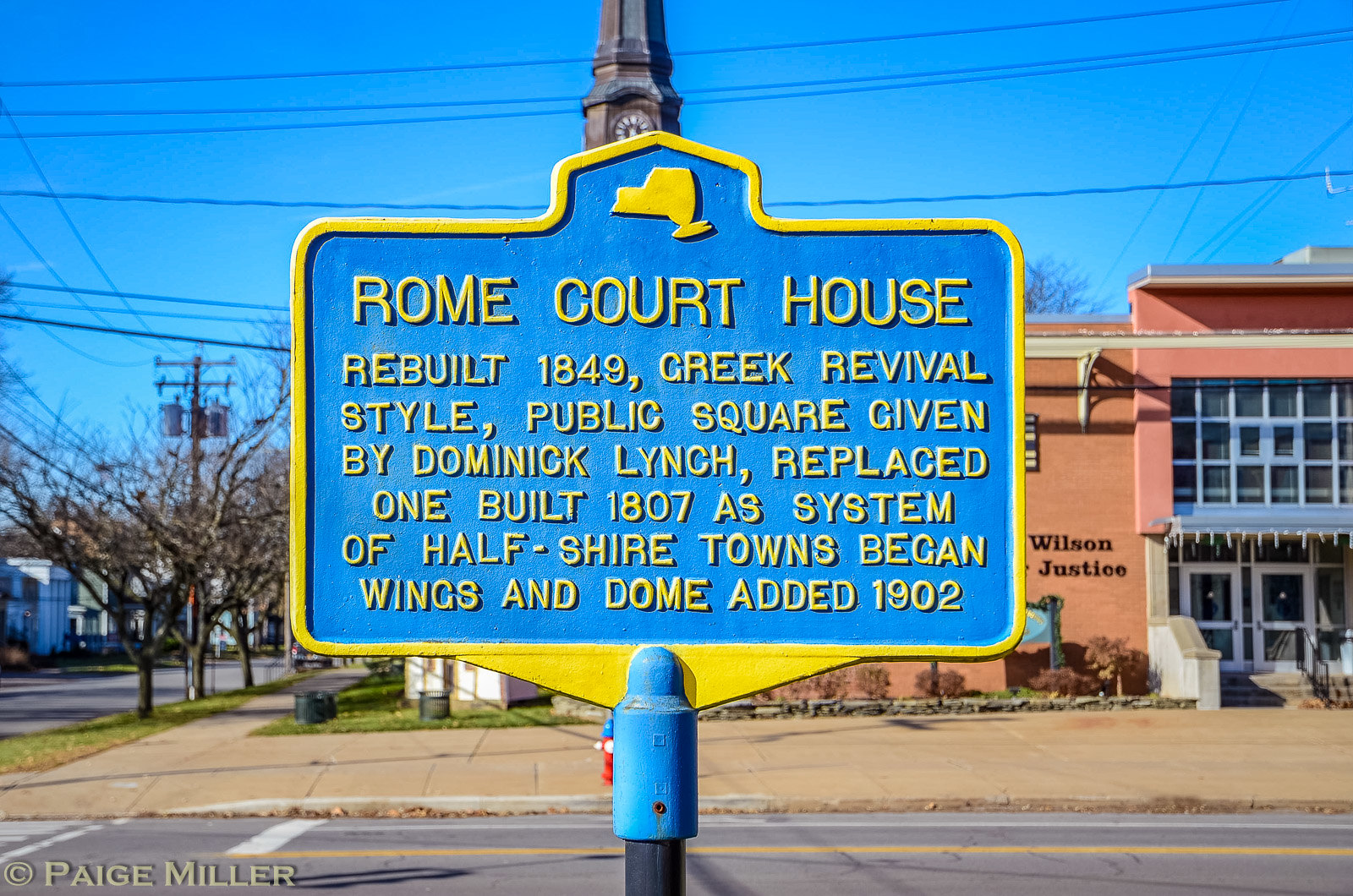The photograph captures a historical marker that you might find on a street pole around a city. The sign is primarily blue with yellow text and outlines, and it features a small icon of the state of New York at the top, also in yellow. The detailed inscription on the sign reads: "Rome Courthouse, Rebuilt 1849, Greek Revival style, public square given by Dominic Lynch, replaced one built 1807, a system of half-shire towns, began, wings and dome added 1902." 

In the background, you can see a road and across the street stands a two-story red brick building. Part of the text on the building is visible, reading "Wilson Justice," suggesting it's a public building likely associated with the courthouse described on the marker. The photograph effectively connects the historical significance of the sign with the courthouse in the background.